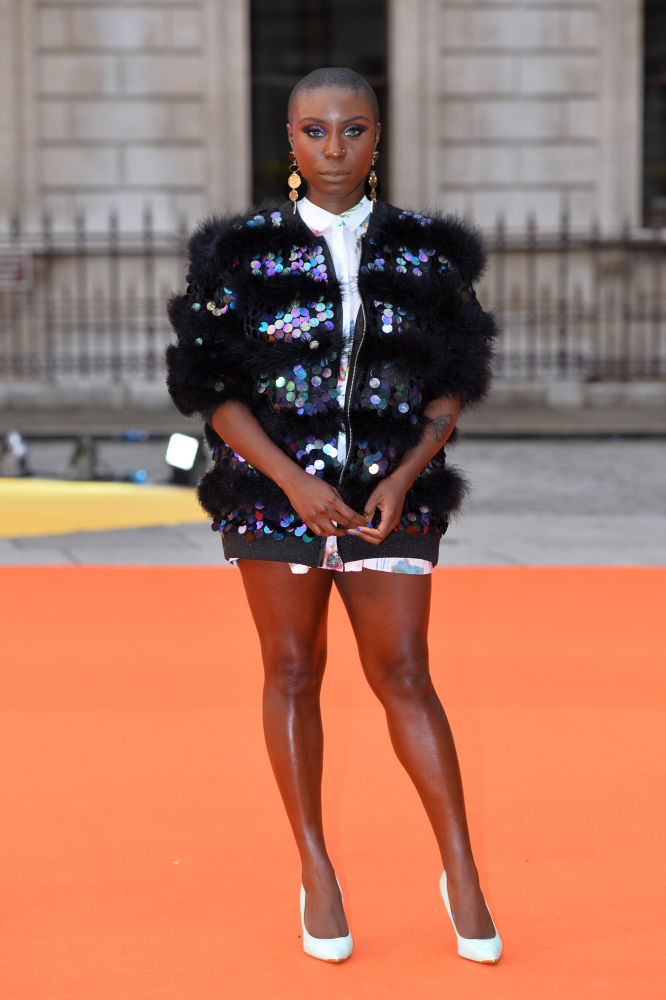The photograph captures a striking image of an African-American woman standing confidently on an orange carpet, set against a grayish-white stone building with black windows and a black fence. Her short, shaved dark hair complements her serious yet captivating expression, as she gazes directly at the camera. She sports a small nose piercing and wears vibrant purplish eye shadow. The woman is adorned in long, round gold earrings that dangle gracefully. Her outfit consists of a white collared button-down shirt, partially obscured by a dazzling black coat. This coat, embellished with large iridescent sequins and fur, features short sleeves that either reach or are rolled up to her elbows and falls to her hips, possibly covering a very short skirt or dress. She completes her ensemble with chic white pumps. The image is vivid and clear, with a bright outdoor setting enhancing the visual details.